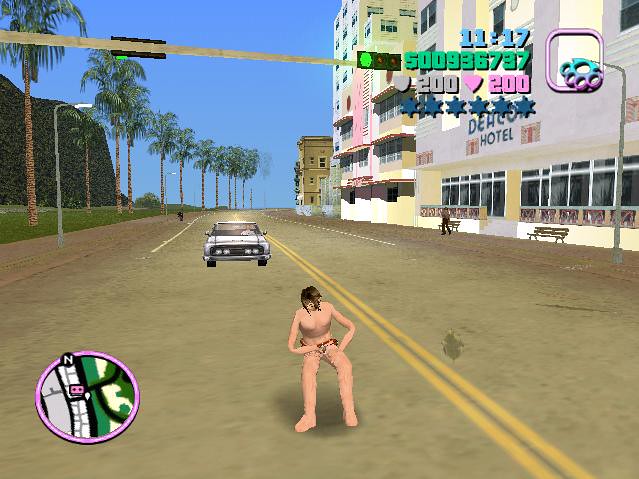This color screenshot is from an older, low-poly Grand Theft Auto game with heavily pixelated graphics, likely at least 15 years old. The scene depicts a nearly naked character, dressed only in underwear, standing in the middle of a city street as a white car approaches from behind in the same lane. The left side of the street is lined with a green hill and numerous palm trees, while the right side features city buildings, including a hotel and what could be apartments or commercial buildings. The game interface displays various statistics: in the bottom left corner, there is a circular map inset; the top right corner shows a pair of brass knuckles with the numbers "11 17 5 0 0 9 3 6 7 3 7," a shield icon and a heart icon both marked "200," and six blue stars.